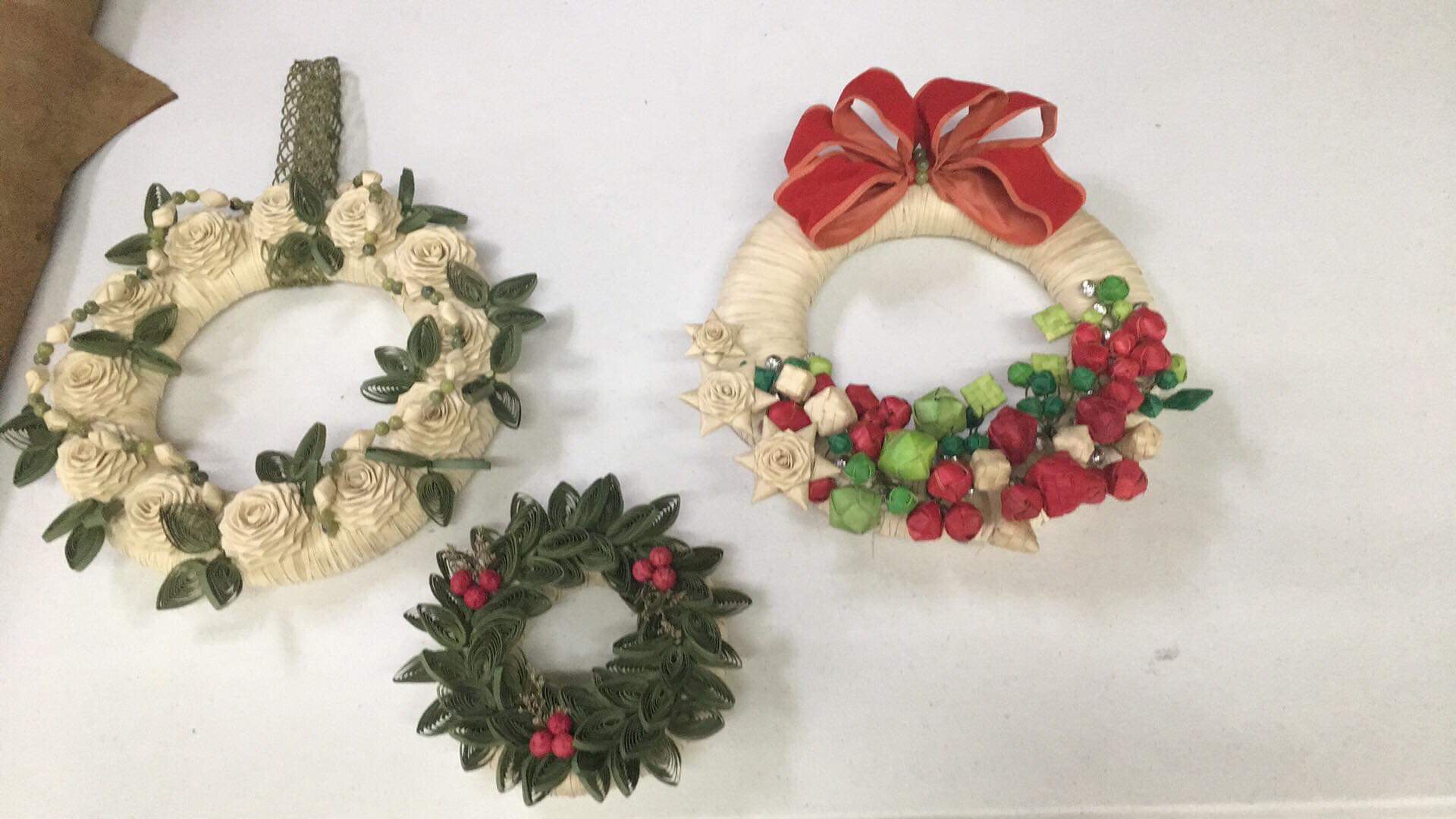This is a photograph featuring three Christmas-themed wreaths arranged on a white background. The largest wreath, positioned slightly to the right, is predominantly cream-colored with an intricate floral design of white roses and features a decorative mix of red, green, and light green buds around its perimeter. It is adorned with a prominent red ribbon at the top. To the left of this wreath, slightly above midline, is another cream-colored wreath, showcasing white roses beautifully complemented by sage-green leaves. This wreath hangs from a matching sage-colored piece and offers a serene aesthetic with its intricate floral details. The smallest wreath, situated near the bottom left, is green with clusters of red holly berries accentuating its simple yet festive design. Its arrangement of three sets of three red berries gives it a classic holiday vibe, reinforcing the overall festive theme of the display.